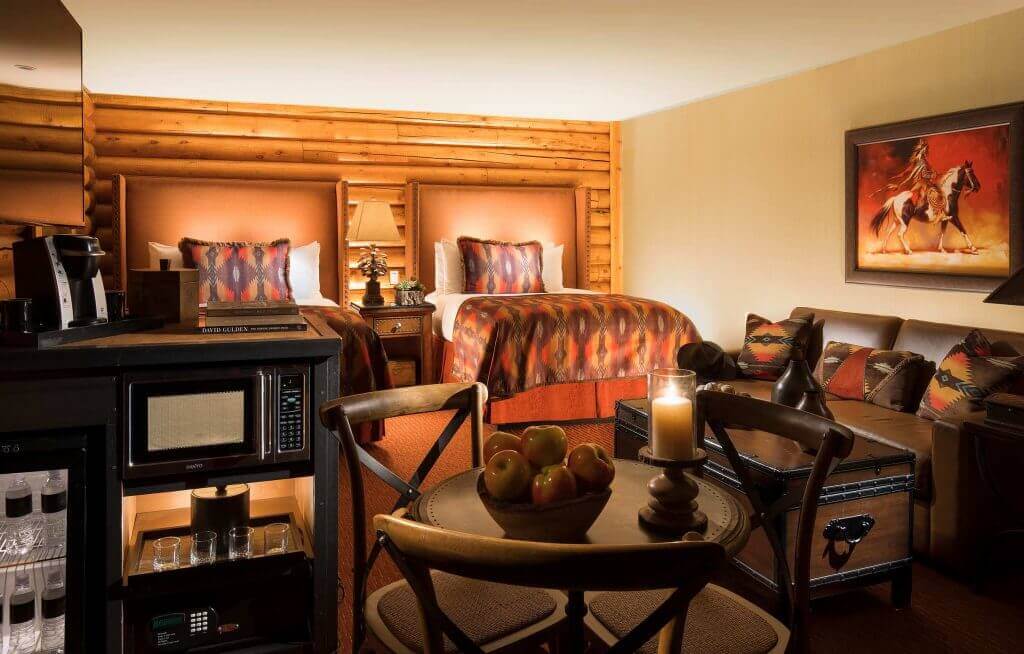This image showcases an intricately furnished interior room, possibly the living room of a home or a hotel suite. The back wall is adorned with elaborate woodwork and features three built-in beds, each separated by a nightstand. The beds are each dressed with ornate yellow and black pillows, prominently featuring a cross in the center. 

To the right of the beds, there's a brown leather couch, also adorned with similar ornate pillows. Hanging above the couch is a painting of a man on horseback, set against an orange background and framed in brown.

In front of the couch, there’s a highly detailed coffee table that resembles a chest, topped with a brown statue. Moving upward in the image, there’s a small dining table with a wooden top, accompanied by three chairs. The table is decorated with a candle on a wooden base and a bowl of various fruits.

To the left of this dining setup, a microwave and a small refrigerator are visible. The refrigerator, loaded with several bottles of water, is surmounted by what seems to be a Keurig-style coffee maker.

This exceptionally furnished room, with its extensive furniture and refined decor, gives the impression of being part of an upscale hotel suite.